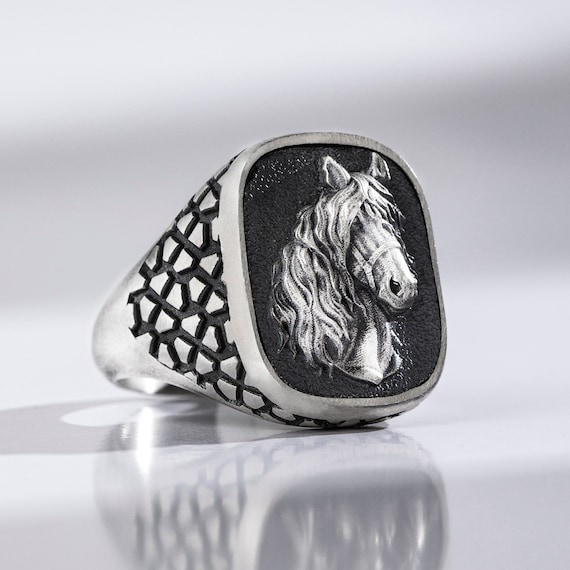The image features a detailed close-up of a silver ring on a light gray, almost whitish background, with a reflection that doesn't reveal much about the surface it rests on. The ring itself has a rectangular shape with elegantly curved sides, and the background within the ring's face is black, showcasing the intricate head of a horse adorned with a bridle and a flowing mane. The design appears to be raised or in relief, suggesting the ring could possibly serve as a stamping tool, although it primarily appears to be a piece of fine jewelry. The side of the ring is decorated with a dark geometric or lattice pattern, adding to its sophisticated aesthetic. Notably, a hint of red reflection is visible on the right side of the image, adding a subtle touch of color to the otherwise monochromatic scene.